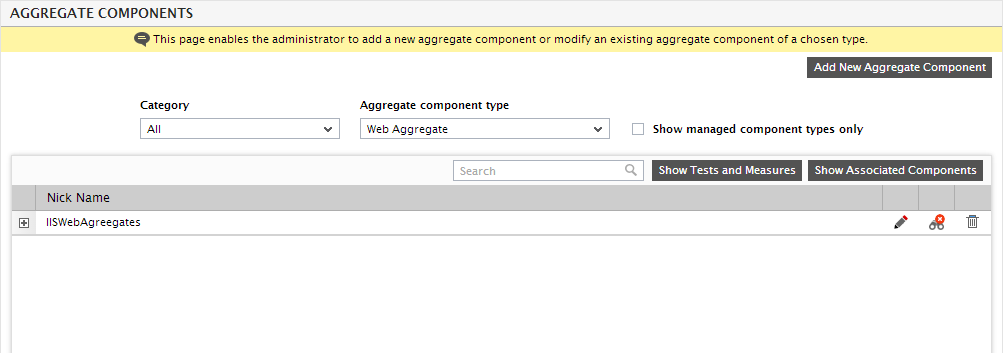The image displays a user interface of a program featuring an "Aggregate Components" section located in the upper left-hand corner. The interface has a gray background with a gray bar across the top, and the text "Aggregate Components" is written in black. Below this header is a yellow warning bar that reads, "This page enables the administrator to add a new aggregate component or modify an existing aggregate component of a chosen type."

Beneath the warning bar, there is a button labeled "Add New Aggregate Component." Following this are two pull-down menus: one labeled "Category" and the other "Aggregate Component." A checkbox is available for users to filter the results to "Show Managed Component Types Only."

Additionally, the interface includes a search bar and two more buttons: "Show Test and Measures" and "Show Associated Components." Below these controls, there is a section currently displaying the nickname "IS Web Aggregates." Next to this label, there is a pencil icon, likely for editing, and another icon with an unclear function. A trash bin icon suggests the option to delete the entry. 

Next to "IS Web Aggregates," a plus box can be clicked to reveal a tree structure or dropdown menu containing additional elements that are currently hidden.